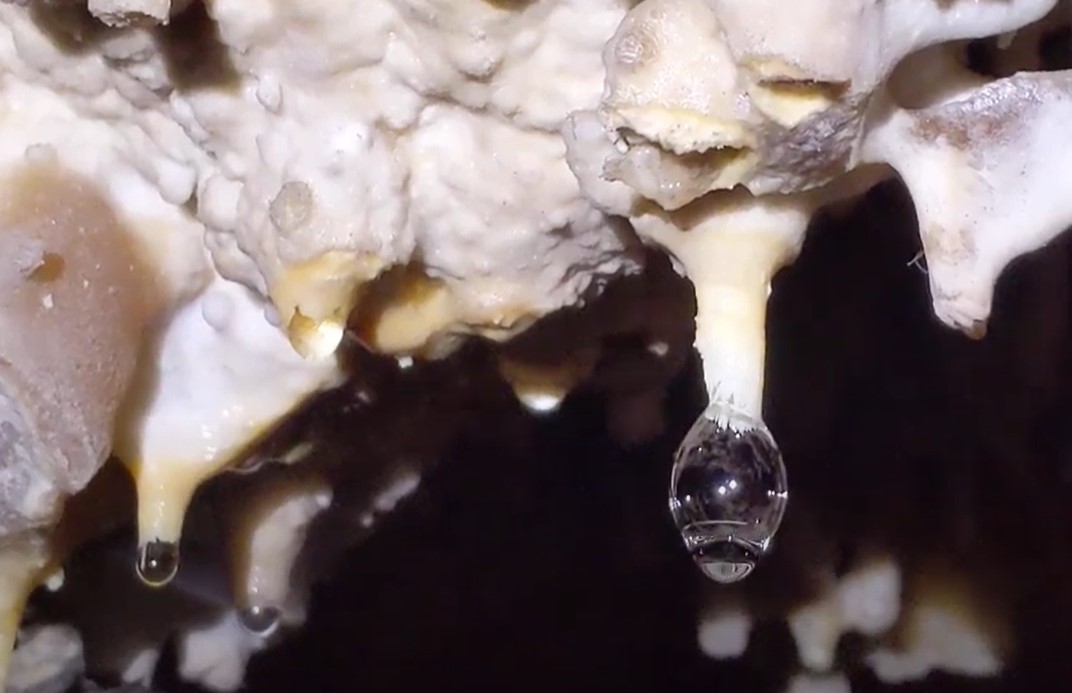The image depicts a dimly lit cave scene with the central focus on the formation of stalactites. Emerging from the ceiling, these rugged and jagged structures are primarily off-white, tan, light gray, yellow, and cream-colored. The intricately textured formations are far from smooth, exhibiting a bumpy and inconsistent appearance. Clear water droplets are visibly dripping from the stalactites, with one of the larger drops forming on the right side, glistening as it hangs precariously. The background of the cave remains shadowy and dark, enhancing the contrast with the well-lit foreground that could be illuminated by a flashlight. The scene hints at a sense of mystery and natural wonder, capturing the delicate interplay between geological formations and the constant motion of water.